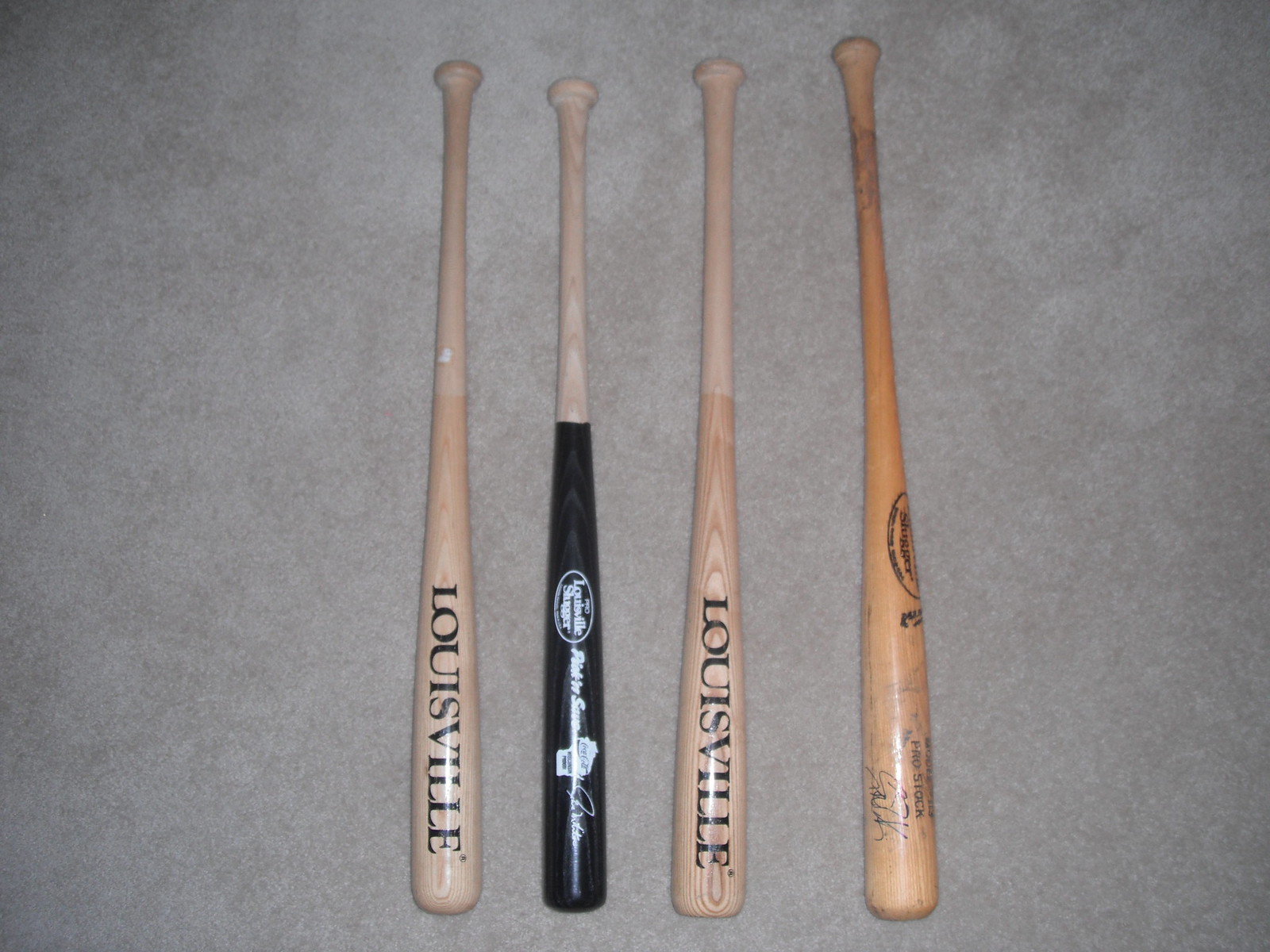This image features four Louisville Slugger baseball bats placed on a light tan shag carpet. Each bat is arranged side by side, with distinct characteristics. The first bat has a light tan wooden handle that transitions into a slightly darker brown top. The second bat has a tan handle and a black-painted barrel with white writing, identified as a Louisville Slugger. The third bat showcases a similar tan handle with a darker brown top and "Louisville" written in black on it. The final bat is a solid honey brown color, a bit longer than the others, with some scuff marks at the end, which might indicate use. This bat also features black writing but no clearly visible brand name. The uniformity and polished look, along with some unique attributes like signatures and dirt marks, highlight both their collectible and practical nature.